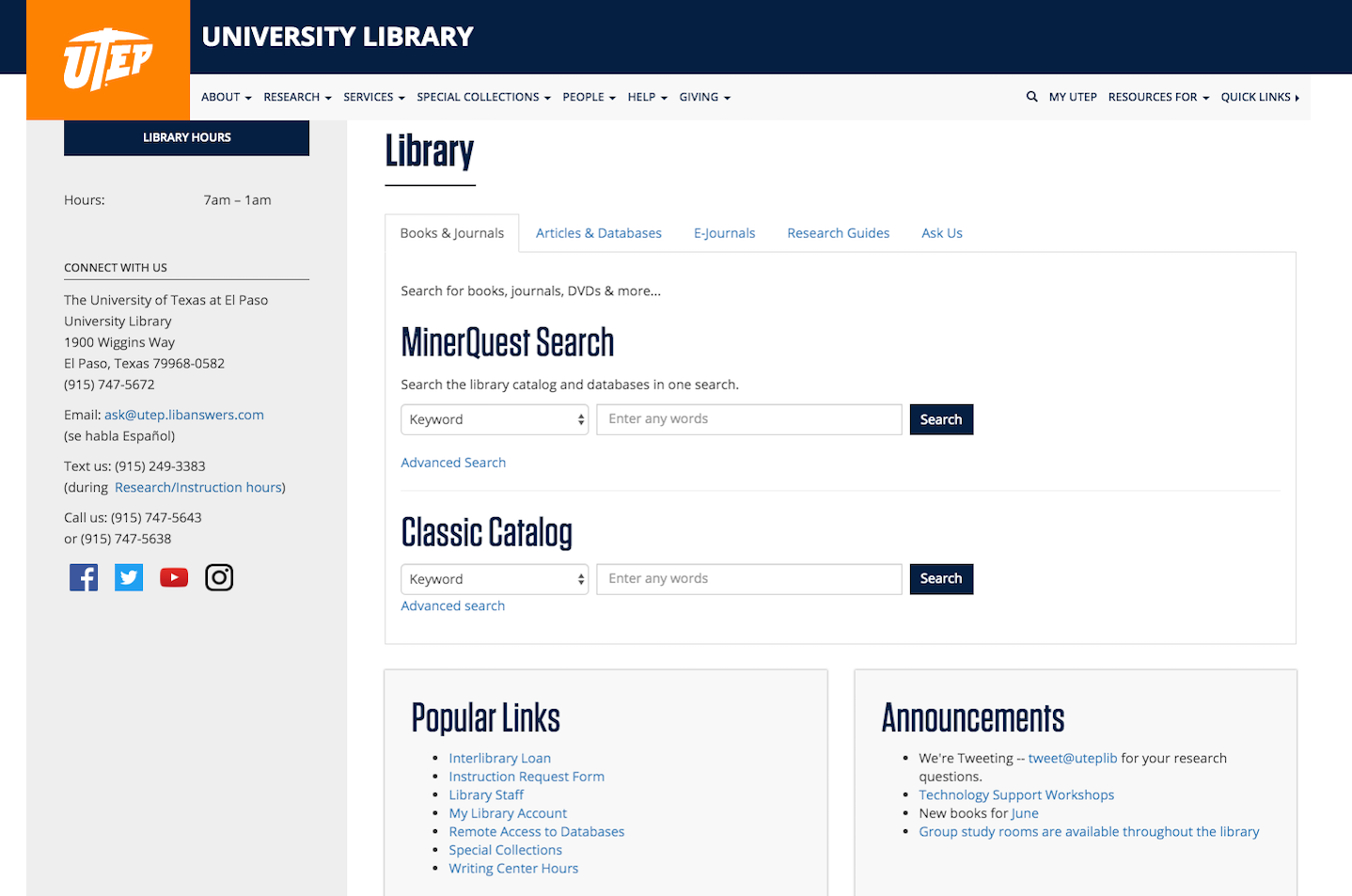In this detailed image captured from the University of Texas at El Paso (UTEP) library website, the focus is on the vibrant and informative layout showcasing various features and resources available to students and visitors. At the top of the page, prominently, the initials "UTEP" are displayed in bold white print against an orange square backdrop. The design of the "T" intriguingly resembles a chisel. Adjacent to this, the title "University Library" is outlined in crisp white letters.

Just below the title, the word "Library" is underlined, followed by navigation options including "MinerQuest Search," a "Classic Catalog," and more. On the bottom left, the "Popular Links" section is displayed, providing quick access to commonly used resources, whereas the "Announcements" section is situated on the right, keeping visitors updated with the latest news and information.

Continuing down the left side, there's a detailed section listing the library hours from 7 a.m. to 1 a.m. Additionally, it encourages connectivity with the library through various means. The address is provided as 1900 Wiggins Way, El Paso, Texas, accompanied by the zip code, phone number, and email address. There's also a note indicating "Se habla español," welcoming the Spanish-speaking community.

For further assistance, it offers a "Text Us" feature with a specific number available during research instruction hours, and multiple contact numbers for phone inquiries. The bottom part of the image includes icons linking to the library's social media pages on Facebook, Twitter, YouTube, and Instagram, facilitating easy access to their online presence.